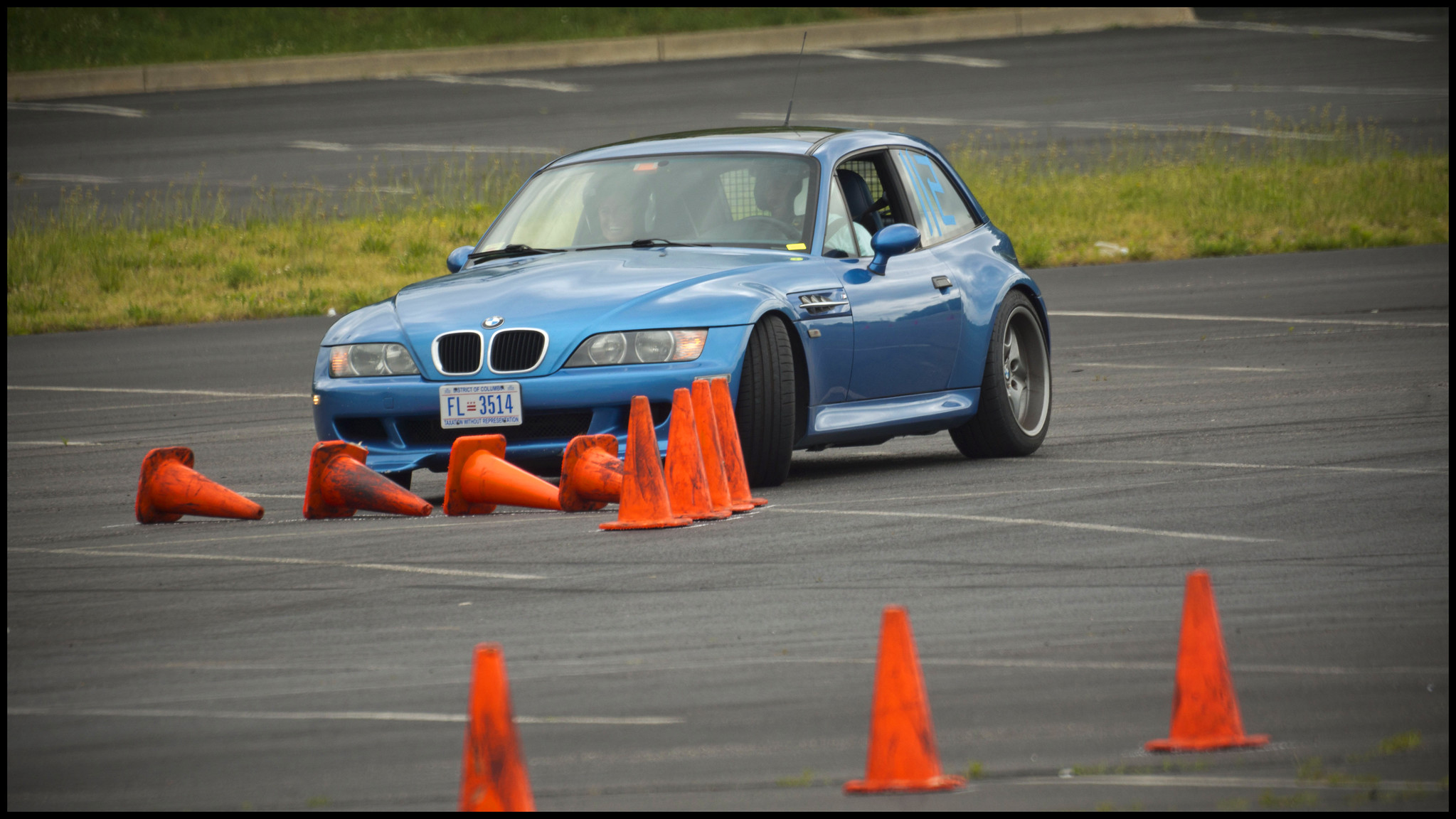This outdoor photograph depicts a blue BMW, possibly a 2019 model from the XB or M-series, situated in a parking lot with weathered black asphalt and faint white diagonal lines indicating parking spaces. Prominently in the foreground are three orange plastic traffic cones, visibly dirty and scuffed black. The focal point, the blue two-door car, has its driver’s side window rolled down, revealing two individuals inside: the driver, who is wearing a seatbelt over the left shoulder and appears focused, and a smiling passenger. The car's front license plate reads "District of Columbia, FL-3514."

Ahead of the vehicle sit seven additional orange traffic cones, four of which have toppled over while three remain upright, similarly dirty and scuffed. The blue car's wheels are turned towards the left of the image, showcasing black tires with large silver rims. The car features three sets of lights on the front, each with three bulbs, and its indicators are illuminated in orange. A black grille with a BMW logo completes the front facade.

In the background, a strip of green grass separates this section of the parking lot from another paved area, beyond which more grass and a concrete curb are visible. The rear driver's side window displays what appears to be the number "112," possibly as part of a track or training session layout. This setting, with scattered and overturned cones, suggests a practice course or driving test being undertaken.